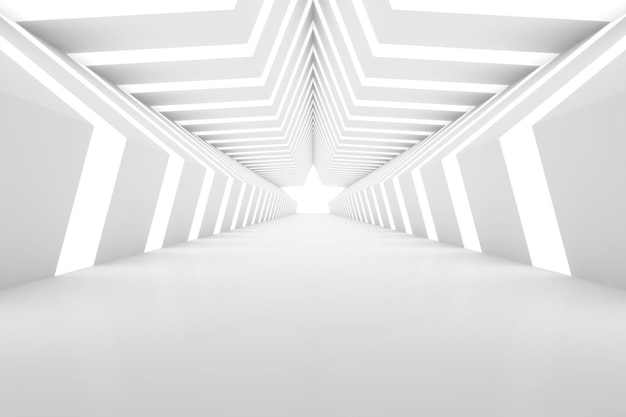The image features a meticulously designed backdrop, reminiscent of a music video or potentially a digitally generated scene. The setting appears to be a long, tunnel-like space adorned with a starry theme. The background is predominantly silver, interspersed with bright white lights that create an illusion of stars shining through. These lights are spaced approximately a foot apart, contributing to the overall luminosity and ethereal feel of the scene.

The tunnel extends straight ahead, leading the eye towards its end, where a half-star structure prominently rises. This star figure, seemingly the focal point and intended "end goal" of the scene, stands at an estimated height of six and a half feet. This elaborate setup evokes the ambiance of a grand music video stage or a celebratory tunnel through which sports teams might emerge before a high-stakes championship game. The intricate details and the strategic placement of lights give the entire image a dynamic and captivating appearance.